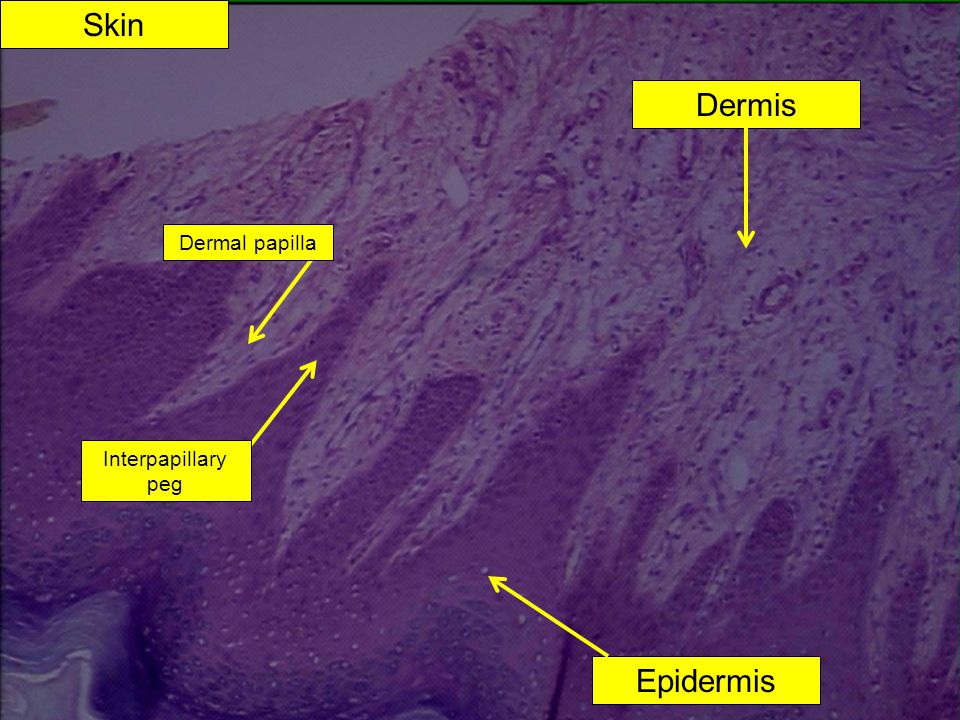This detailed image depicts a highly magnified view of skin, rendered in various shades of purple rather than natural skin tones. The image, which takes up the entire frame, is annotated with several yellow boxes containing dark blue or black text to identify and describe different skin structures. 

In the upper left, a yellow box with dark blue or dark purple text labels the image as "skin." Additional yellow boxes with arrows point to specific areas: 

- The upper right section features a box labeled "dermis," with an arrow directing downward.
- Below and to the left is another box labeled "dermal papilla," with an arrow pointing to the bottom left.
- Further down is the label "interpapillary peg," with an arrow extending from the top right of the box.
- In the bottom right corner, another yellow box labeled "epidermis" has an arrow pointing to a small white speck on the skin.

The annotations serve to highlight and educate the viewer on the various components of the skin, making the image a valuable learning tool despite its unconventional color palette.